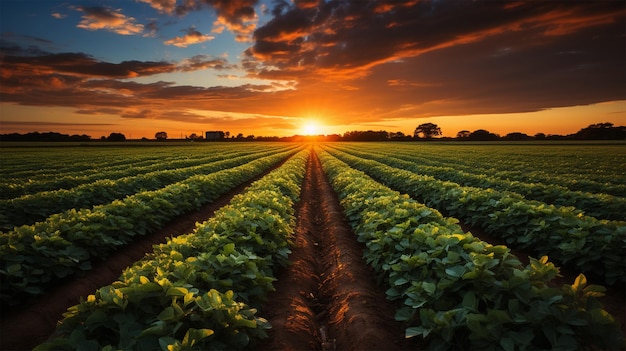A serene sunset casts a golden hue over a meticulously maintained crop field, extending into the distance toward the horizon where the sun is halfway set. The lush green rows of what appears to be potato plants stretch out in neat, weed-free furrows of rich, dark brown soil. The lines of the crops seem to converge at the setting sun, creating a deeply picturesque vista. Above, the sky transitions from a darkening blue at the top to a captivating blend of rosy red, pink, and orange hues, with wispy clouds illuminated by the fading light. Silhouettes of distant trees and farm buildings add to the tranquil rural landscape, though the scene's almost perfect, well-manicured appearance evokes a sense of being either heavily edited or unreal. The overall impression is one of quiet beauty and meticulous care, as each detail in the field reflects a sense of dedication and serenity, enhanced by the elegant play of light and shadows at this magical time of day.